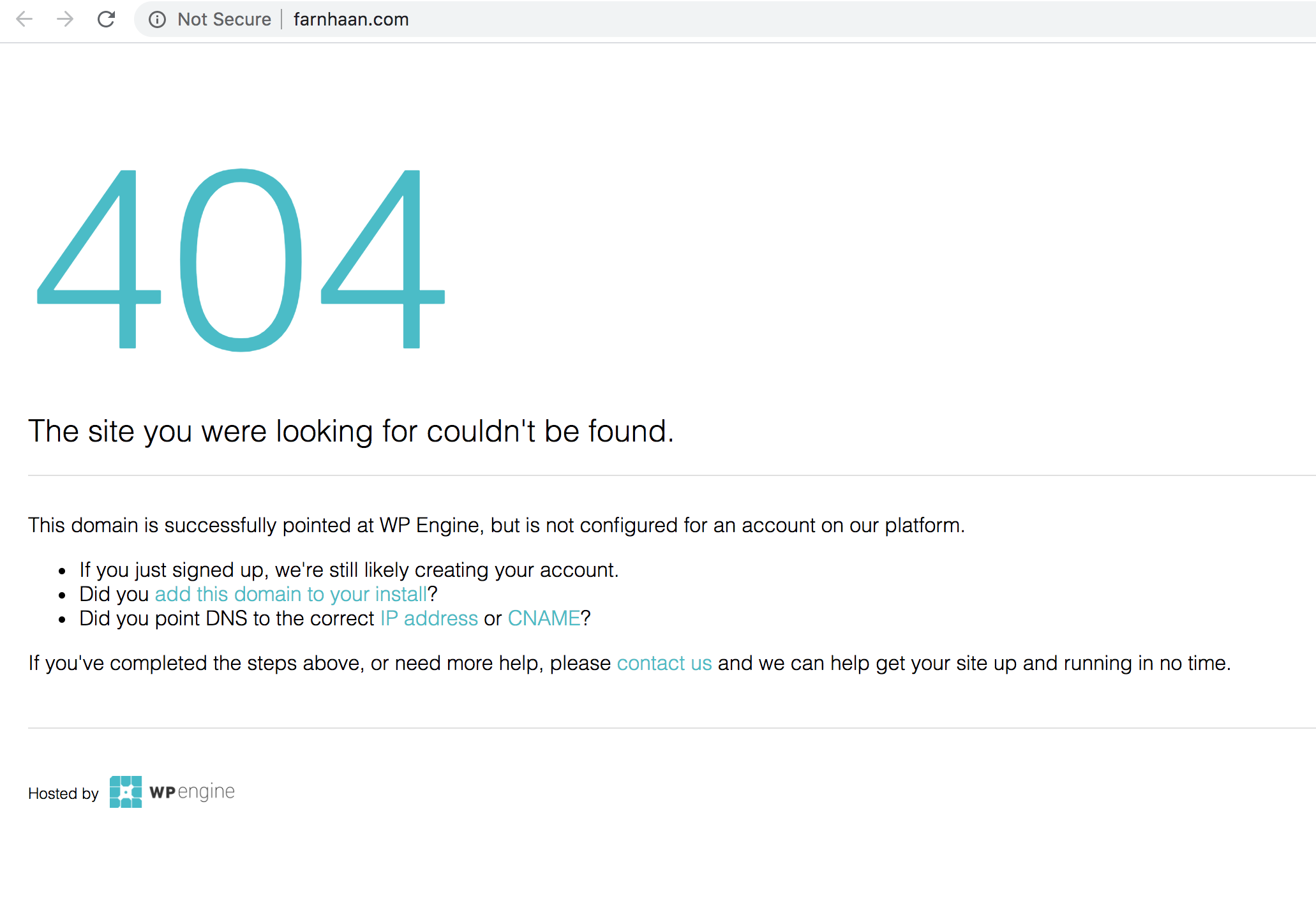The image displays a common error message encountered online. Prominently featured at the top in large teal letters is the number "404." Below that, in smaller black print, the message reads: "The site you were looking for couldn't be found." Beneath this, additional text explains: "This domain is successfully pointed at WP Engine but is not configured for an account on our platform. Did you add the domain to your install? Did you point DNS to the correct IP address or CNAME?"

The error message continues with instructions for further assistance: "If you completed the steps above or need more help, please contact us." The phrase "contact us" is formatted as a clickable blue hyperlink, indicating users can click on it for additional support to get their site operational. At the bottom of the image, there's a teal square with the text "Hosted by WP Engine," signifying the web hosting provider.